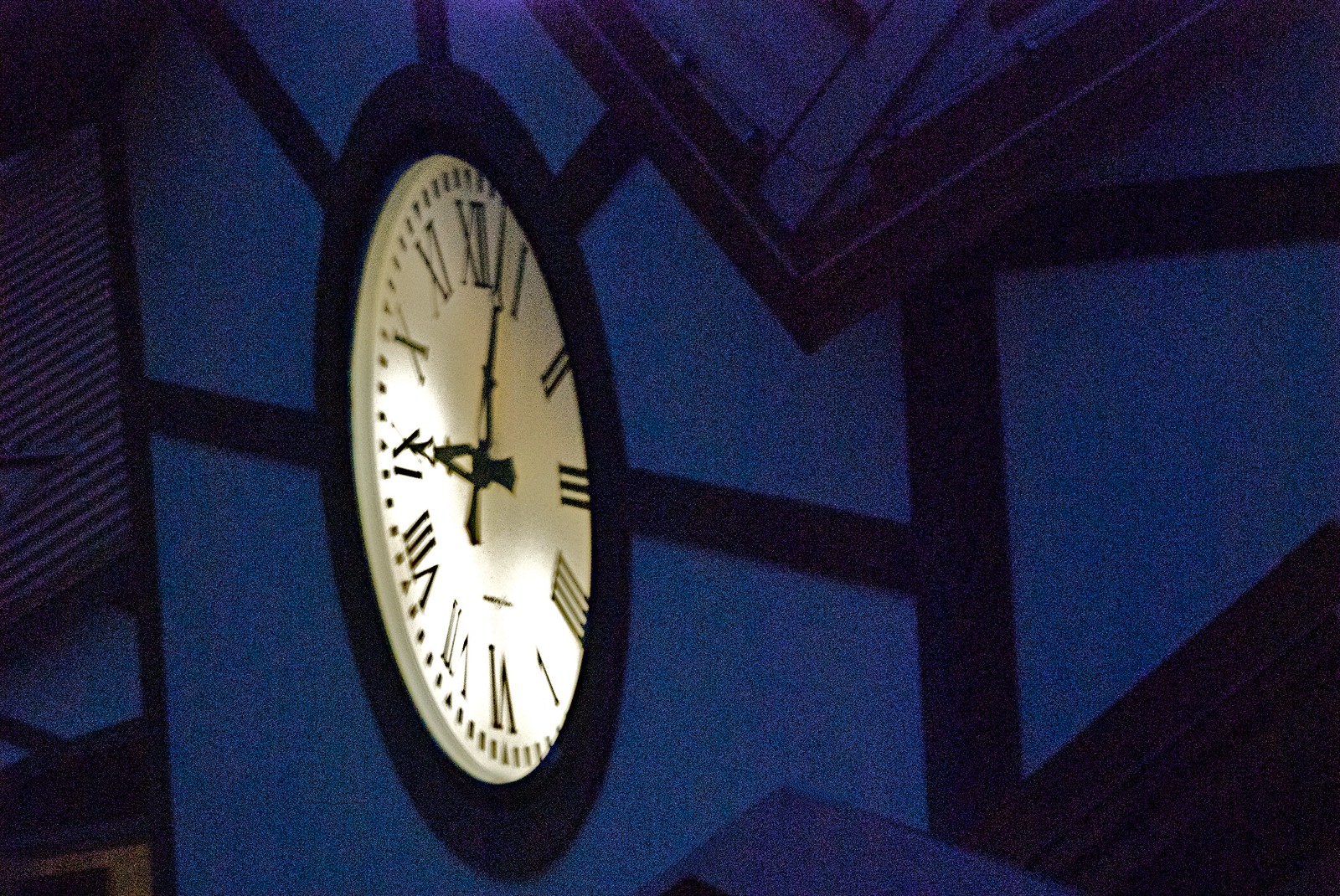The photograph depicts a large clock prominently displayed on the exterior wall of a medium blue clock tower, accentuated with dark blue decorative perimeter lines and panels. The image, slightly wider than it is tall, captures the clock at a peculiar angle from a position slightly higher and to the side, making the face appear somewhat oval due to the perspective. The clock has a white face illuminated from behind, clearly showing the time as 9:02 p.m. The numbers are traditional Roman numerals from I to XII, and two uniquely shaped black hands indicate the time. The tower itself features a mix of structural elements, including sections resembling half-timbered designs and shingle-like wood panels near the top left corner. The surrounding night sky is very dark, possibly contributing to the overall low resolution of the image. You can also glimpse parts of a roof, suggesting the structure's architectural complexity.